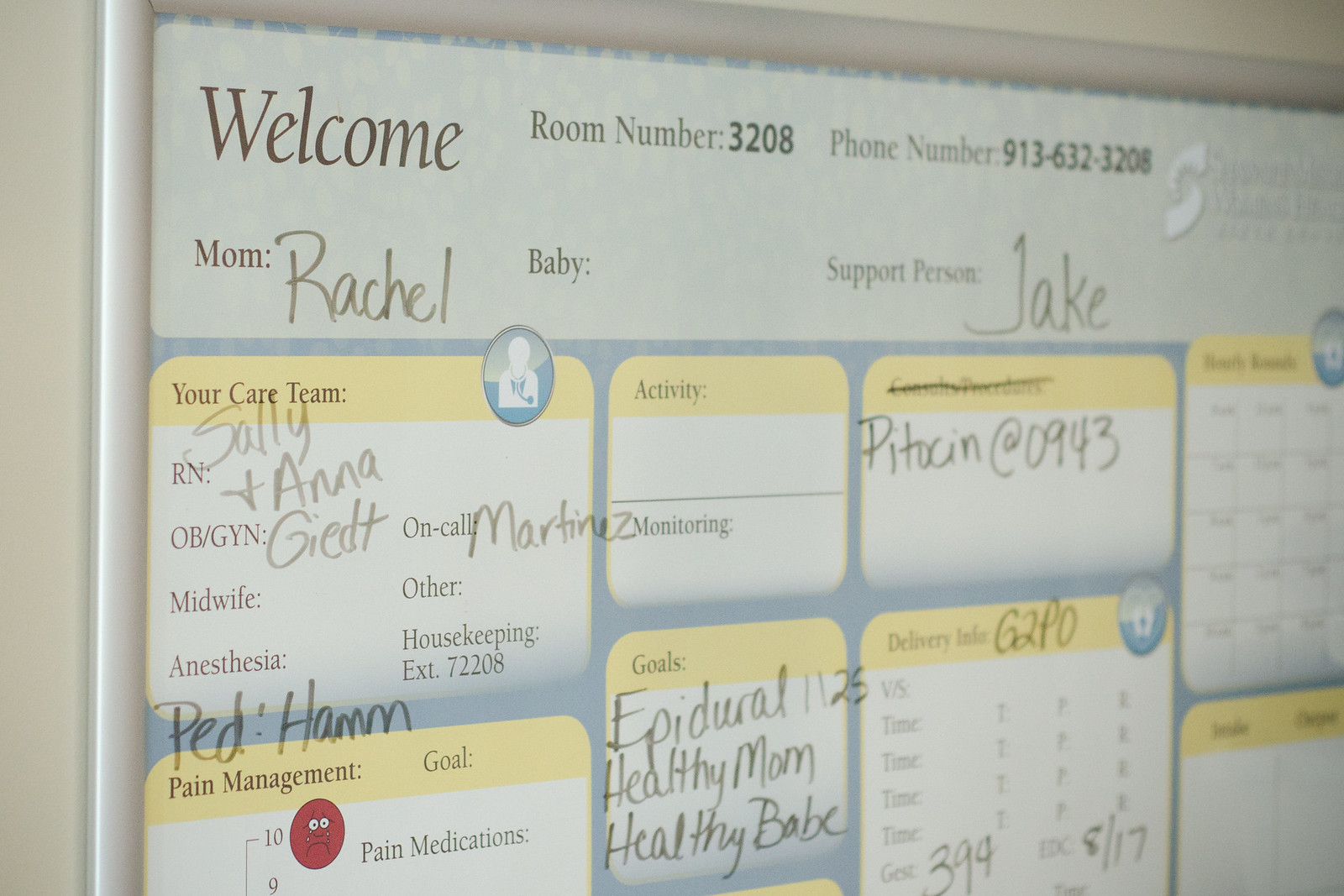The image shows a detailed whiteboard posted in hospital room number 3208, providing crucial information for the medical staff. At the top, it says "Welcome" in black letters, followed by the room number and a phone number. The board identifies the mom as "Rachel" and leaves the “Baby” section blank, indicating the baby’s name hasn’t been filled in yet. The support person is listed as “Jake.” 

The whiteboard is divided into various sections filled out with handwritten information. The left section, labeled "Your Care Team,” includes names and titles for the RN, OBGYN, and other critical team members but leaves some roles such as midwife and anesthesia blank. Adjacent to this section is a box for "Pain Management," where a pain level of 10 is noted, indicating severe pain. Below this section, there are listings for different medications like "Pedicodin at 0943" written down.

To the right of the Care Team section, boxes labeled "Activity" and "Monitoring" are currently blank, while further to the right is a partially visible calendar. Another box, titled "Goals," lists specific objectives such as "epidural," "healthy mom," and "healthy babe." Below the goals section is a "Delivery Info" area, with specifics like "GEST: 39.4" and a date of "8/17."

Overall, the whiteboard is bordered by a silver frame and spans to the edges of the image, indicating a systematic and organized approach to patient care in what appears to be a maternity ward.